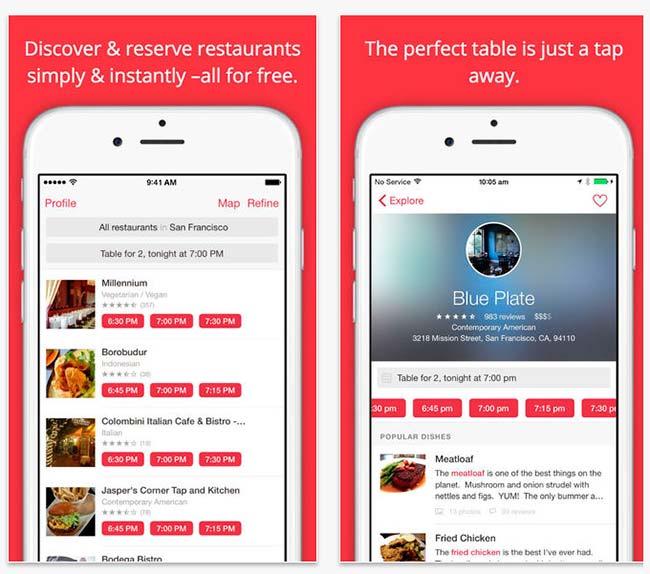Introducing an app store mockup featuring a sleek white iPhone showcasing a reservation platform for restaurants. This virtual model highlights comprehensive app functionalities with a seamless and visually appealing interface.

At the top left in a vivid red section, the text reads: "Discover and reserve restaurants simply and instantly—all for free." Below, a webpage is displayed within the smartphone screen. The status bar indicates a full Wi-Fi signal, the time as 9:41 AM, and a fully charged battery symbol. The menu bar under the status indicates "Profile" in red text on the left, flanked by "Map" and "Refine" options on the right.

The primary interface is segmented into multiple actionable sections:
1. Two dark gray rectangles: 
   - The first labeled "All Restaurants" with "San Francisco" in gray text.
   - The second addressing a search query: "Table for two, tonight at 7 PM."

2. A series of restaurant listings, each with a dedicated button for reservation times:
   - "Millennium": Featuring an elegant white décor, it is a vegetarian and vegan restaurant with 357 reviews. Reservation times: 6:30 PM, 7:00 PM, 7:30 PM.
   - "Borobudur": An Indonesian eatery with 328 reviews and a rating of 3.2 out of 5. Reservation times: 6:45 PM, 7:00 PM, 7:15 PM.
   - "Colombini Italian Café and Bistro": Displaying a snippet, it has 18 reviews and a 4 out of 5 rating. Reservation times: 6:30 PM, 7:00 PM, 7:30 PM.
   - "Corner Tap and Kitchen": Featuring a burger with lettuce and cheese, it is described as Contemporary American with 78 reviews and a 3.3 out of 5 rating. Reservation times: 6:45 PM, 7:00 PM, 7:15 PM.

The screen's lower section iterates the search for a "Table for two, tonight at 7 PM" in a light gray box. Popular dishes from the highlighted restaurants include:
   - "Meatloaf," celebrated as "one of the best things on the planet," garnished with green vegetables.
   - "Fried Chicken," lauded as "the best I've ever had," served with a golden crust and dipping sauce.

The right side of the display indicates a different time (10:05 AM) and a battery icon now in green, with a "No Service" notice despite full Wi-Fi bars. A black arrow points right, accompanied by a gray Bluetooth symbol. A red header prompts: "The perfect table is just a tap away."

In a blue profile section, the highlighted restaurant "Blue Plate" boasts a panoramic view of green trees through a window, holds a 4.3 out of 5 stars rating with 963 reviews, and lists its location in San Francisco, CA. Three out of four dollar signs indicate its pricing level description.

This detailed, refined mockup offers a clear, user-friendly preview of a restaurant reservation app, emphasizing the ease and efficiency of booking dining experiences.